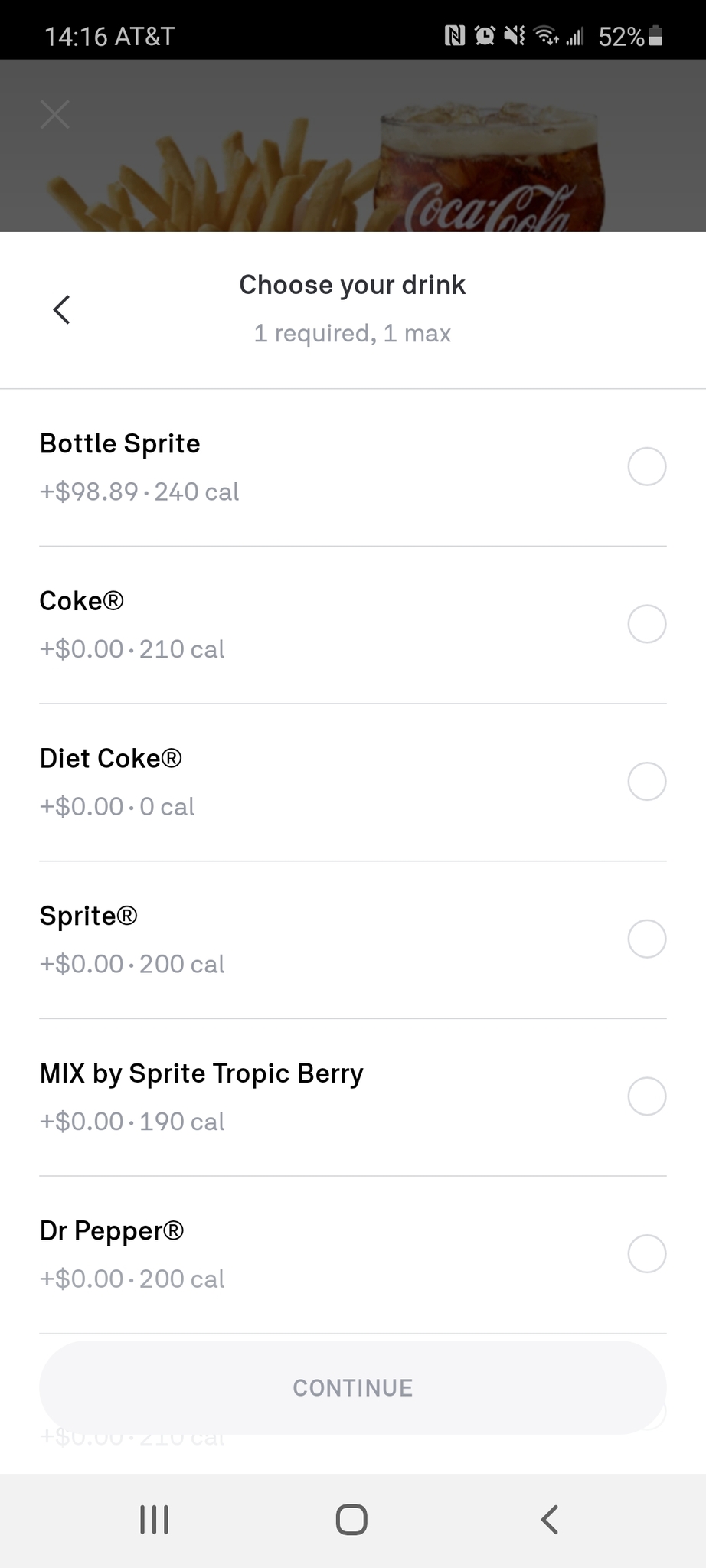This is a detailed screenshot of a smartphone display.

At the top, the time reads 14:16 and the network carrier is indicated as AT&T. To the right, several icons are visible, including an alarm, internet signal bars, and a battery indicator showing 52%.

Just below the top row, there is an image section displaying the top part of French fries and a glass with the "Coca-Cola" logo, containing a caramel-colored soda with slight foam at the top.

Beneath this image, a darkened section reads: "Choose your drink," followed by the instruction, "1 required, 1 max." There is a carrot symbol (">") pointing to the left, and the first drink option listed is:
- "Bottle Sprite, +$98.89, 240 calories," with an unselected circle next to it.

The subsequent drink options are listed as follows:
- "Coke®: +$0.00, 210 calories," with an unselected circle.
- "Diet Coke®: +$0.00, 0 calories," with an unselected circle.
- "Sprite®: +$0.00, 200 calories," with an unselected circle.
- "Mix by Sprite Tropic Berry: +$0.00, 190 calories," with an unselected circle.
- "Dr. Pepper®: +$0.00, 200 calories," with an unselected circle.

At the bottom of the screen is a "Continue" button. Below this, there are three icons representing the navigation buttons on an Android phone: three horizontal lines, a square, and a carrot pointing left.

This detailed caption provides a comprehensive overview of the screenshot's contents, ensuring clarity and completeness.